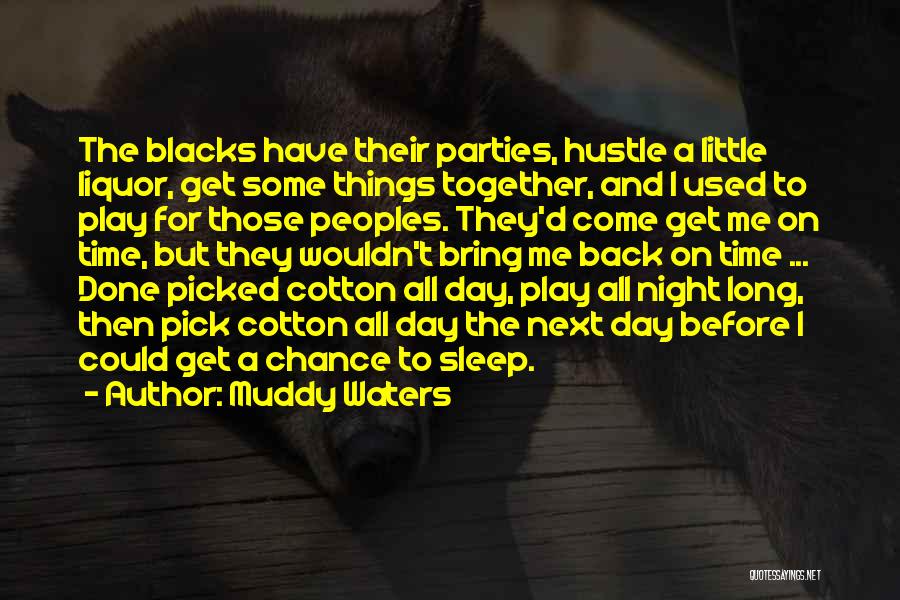The image features a dark and somewhat indistinct background that appears to be a black-and-white photograph of an animal, possibly a dog or a wild animal like a fox, with a bushy tail. The animal seems to be on a wooden porch, adding to the rustic atmosphere. Dominating the center of the image is a bright yellow quote in large text, which reads: "The blacks have their parties, hustle a little liquor, get some things together, and I used to play for those peoples. They'd come get me on time but they wouldn't bring me back on time. Done picked cotton all day, play all night long, then pick cotton all day the next day before I could get a chance to sleep." This quote is attributed to Muddy Waters and is the focal point of the image. In the bottom right corner, in smaller text, it says "quotesaying.net."